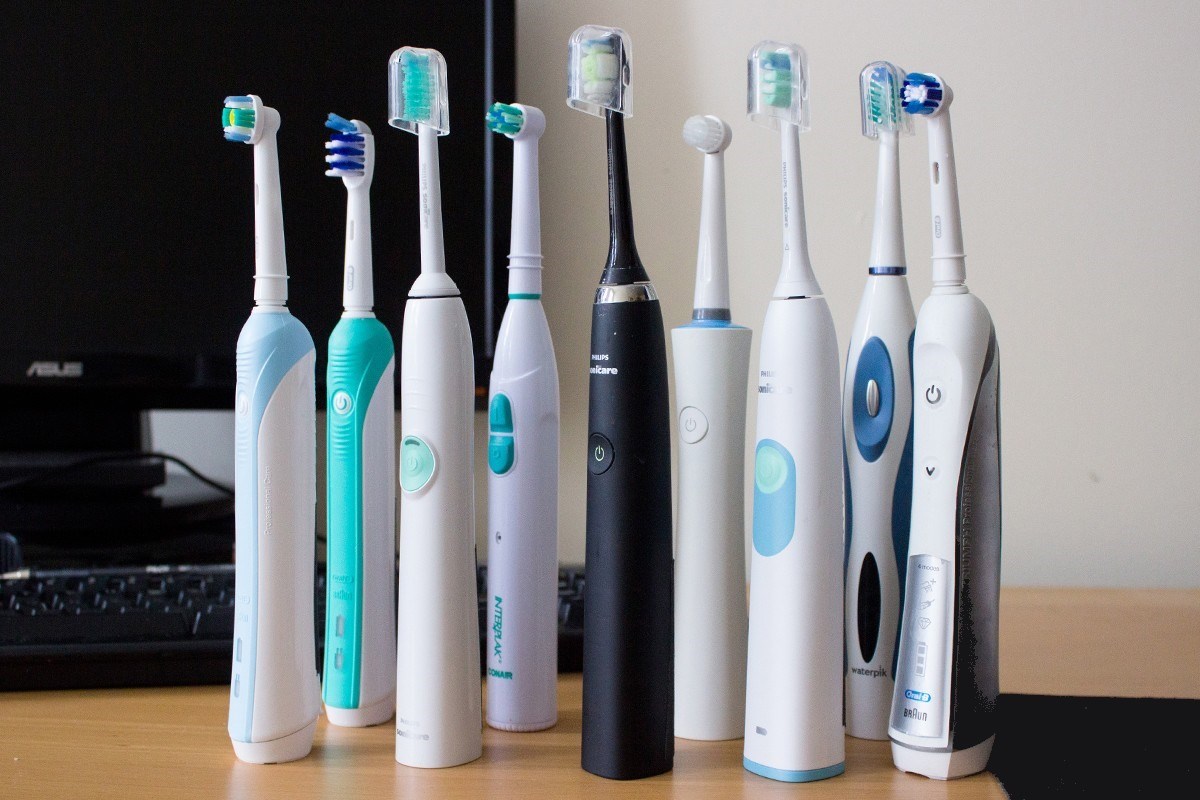In the image, there's a beige-colored white wall in the background and a wooden table or desk in the foreground. On this table, there is a black keyboard and a black Asus computer monitor positioned on the left side. Dominating the scene are nine electric toothbrushes standing on their bases, showcasing a variety of designs and colors, including white, black, light blue, dark blue, turquoise, and gray. Some toothbrushes have caps on their heads while others do not, indicating different types and functionalities.

Four toothbrushes have caps, covering the longer toothbrush heads. The remaining five either have round heads or longer heads without caps. Notably, one toothbrush is black with a silver ring around its neck, adding a distinct contrast to the surrounding primarily white toothbrushes, which display various accents of blue or teal. The toothbrush in the center stands out with its sophisticated black and silver design, while another to the right has a white body with black accents along its sides.

The toothbrushes exhibit a mix of bristle and button colors including teal, green, and blue, providing a visual diversity that suggests different brands and models. Contrary to typical setups, these toothbrushes do not have bases underneath, emphasizing their unique design and making them the focal point of the composition. In the bottom right corner of the image, there's a mysterious black square, the nature of which is unclear but adds an element of intrigue to the scene.